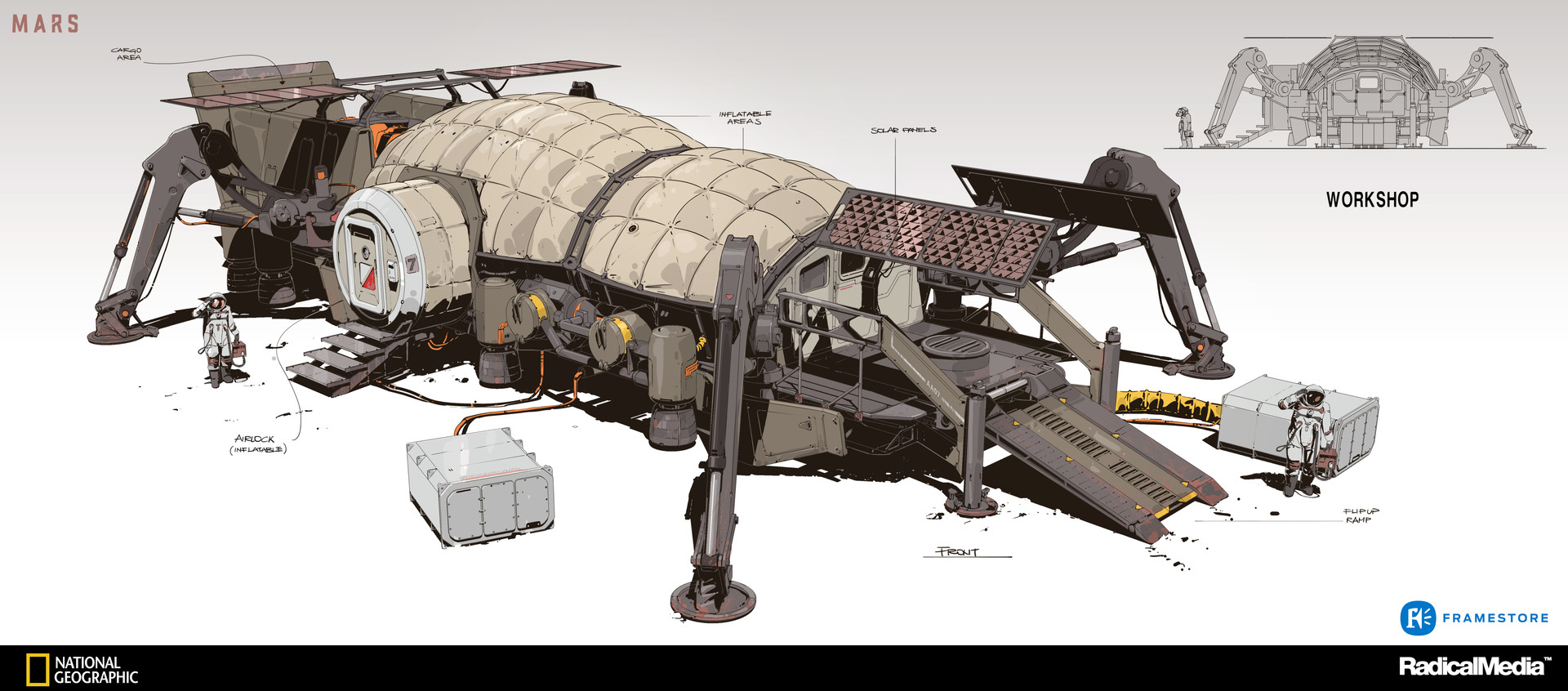This detailed illustration by Oscar Cafaro, featured in National Geographic and Radical Media, depicts a specialized transportation machine designed for use on Mars. The machine's design, reminiscent of an ant or an insect with four sturdy brown legs, combines functionality with a unique aesthetic. Prominent features include solar panels for energy, a long ramp at the front for access, a generator, and a side door with stairs. Two astronauts, dressed in cosmonaut suits with helmets, stand near the machine—one in front and one to the back—indicating human interaction with the transport. Labels on the illustration identify key elements: "Mars" appears in the upper left, "Workshop" alongside a frontal view of the transport is in the upper right, and other features such as an airlock, inflatable areas, and a cargo section are marked. The lower left corner is marked with "National Geographic," confirming the source of this intricate and speculative portrayal of Martian exploration equipment.